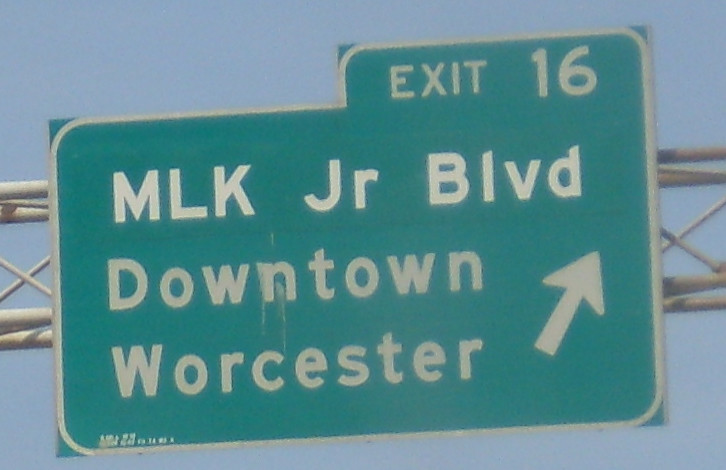The image captures a large green traffic directional sign mounted on a sturdy silver, criss-cross steel frame, likely overhanging a highway, suggesting a close-up, road-level point of view. At the top right corner, the sign prominently displays "EXIT 16" in bold white letters. Directly beneath it, "MLK Jr. BLVD" (an abbreviation for Martin Luther King Jr. Boulevard) appears in a larger, bolder font. Further down, the words "DOWNTOWN WORCESTER" are displayed in a slightly faded white font, concluding with a diagonal arrow pointing to the top right, indicating the direction. The background showcases a relatively clear, blue sky, adding to the overall visibility of the sign's details. The photo's slightly grainy texture suggests it may have been taken from a moving vehicle or through a window.